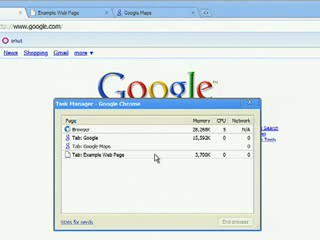The image is a partial, blurry screenshot of a web browser window displaying the Google homepage. The snapshot is notably small, approximately 1.5 inches by 1.5 inches. At the top of the browser, three tabs are visible: one is cut off, another possibly labeled "example web page," and the third is "Google Maps." Central to the image is a dialog box titled "Task Manager - Google Chrome," displaying the memory, CPU, and network details of four browser tabs, including "Google," "Google Maps," "example web page," and another tab. The Google homepage, visible behind the Task Manager, features the word "Google" in its signature colorful text near the top. The browser menu shows several options, including a blurred "shopping" menu and possibly a "more" dropdown. Another tiny detail suggests a menu bar at the top that reads "www.google.com."